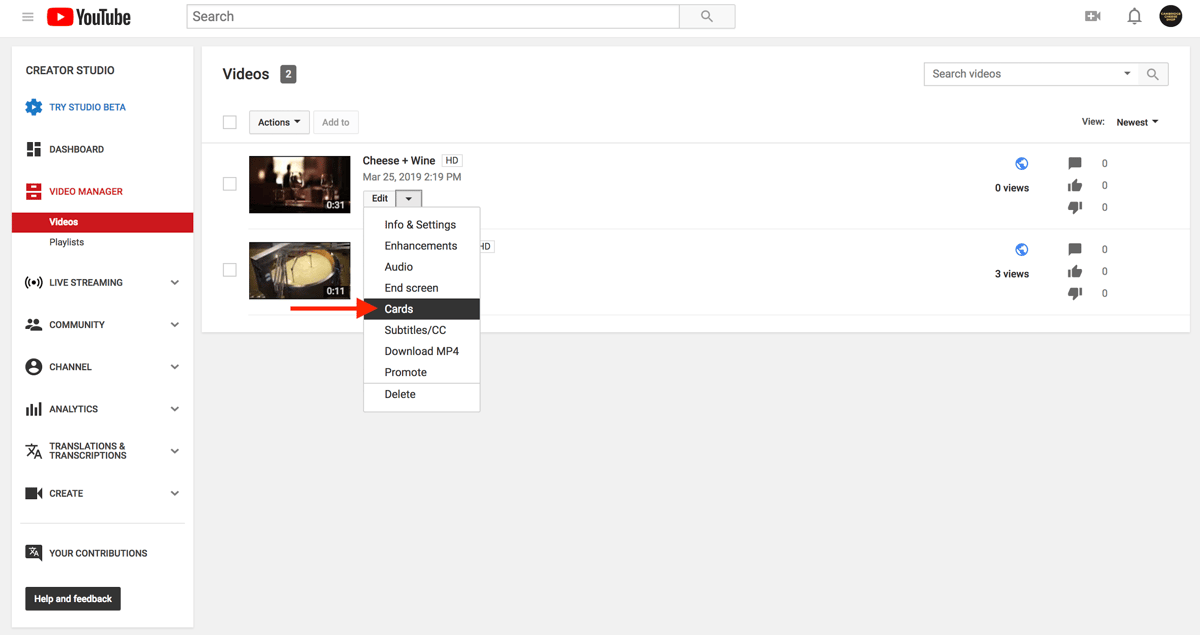The image shows a YouTube interface that appears different from usual, indicating that the user might be signed in to their account. On the left side, there's a pane labeled "Creator Studio," featuring sections such as Studio Beta, Dashboard, Video Manager, Live Streaming, Community, Channel, and Analytics. They are currently in the "Video Manager" section, specifically in a subsection called "Videos."

In the "Videos" subsection, two videos are listed. The first video is titled "Cheese and Wine" and has a duration of 30 seconds. The second video is 11 seconds long, but its title is obscured by a context menu. The "Cheese and Wine" video is in the process of being edited, revealing additional options like Info and Settings, Enhancements, Audio, End Screen, Cards, Subtitles, Download MP4, Promote, and Delete. A red arrow points to the "Cards" option among the settings.

On the right side, the video view counts are visible; the 11-second video has three views, while the "Cheese and Wine" video currently has no views, suggesting it might not be published yet. The interface also displays options to manage Comments, Likes, and Dislikes, hinting at features that allow turning them off.